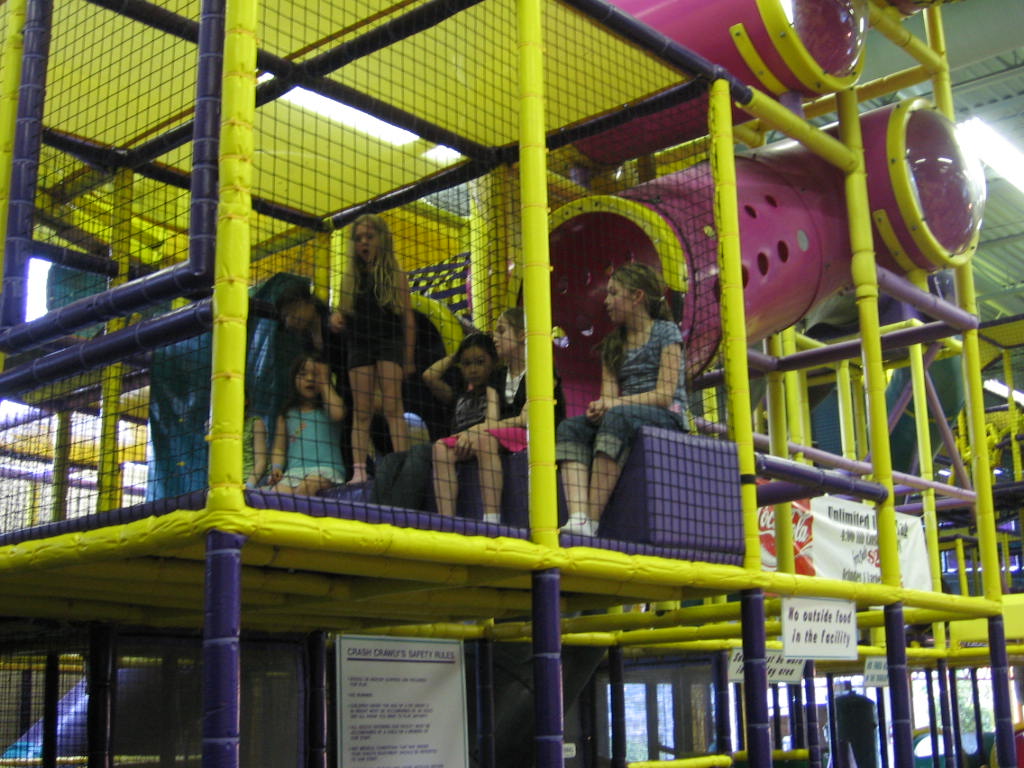The photograph depicts a multi-story children's play area commonly found in large fast-food restaurants or mall play zones. The play structure is constructed with padded yellow and blue framework, and includes various elements such as slides, ladders, tubular slides, bubble windows, and padded sections for jumping, sliding, and climbing. Mesh sides are present for safety, preventing falls. The foreground features several youngsters, possibly around five to eight years old, gathered on the second level beneath a slanted magenta tube with orange rims. Some of these children appear to be seated somberly, with one child standing and another with a hand lifted to their face, possibly crying. The poles of the structure are purple and yellow, and there is a prominent Coca-Cola banner suggesting its location in a kid-friendly fast food establishment.